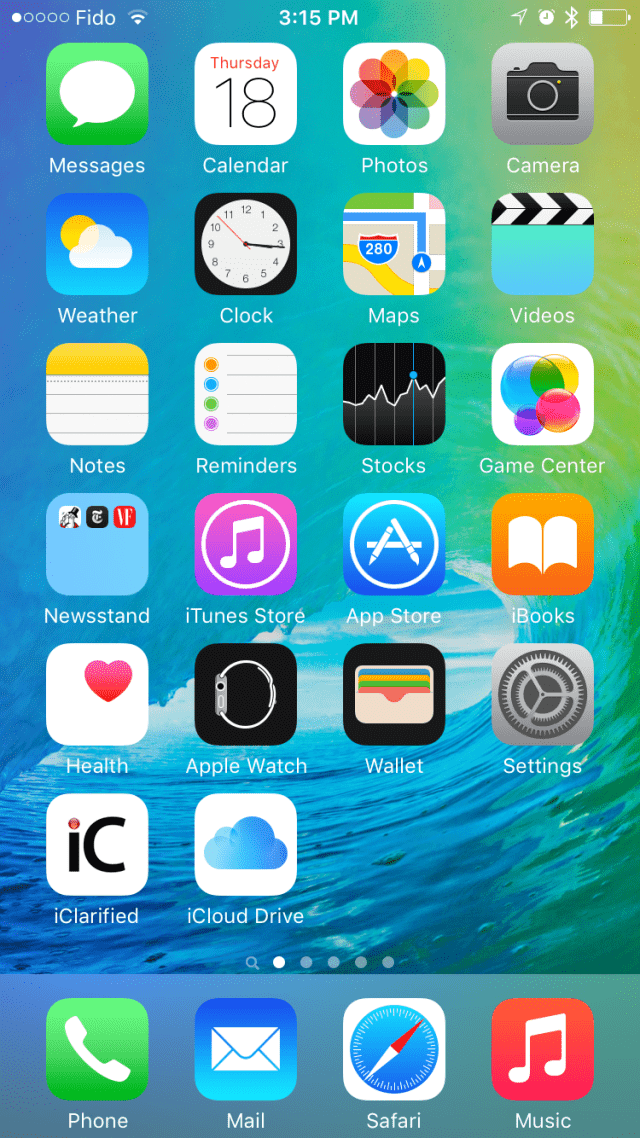The image showcases the homepage of an Apple device, possibly a tablet given the square proportions of the screen. A heading at the top reads "FIDO at 3:15". The homepage features various app icons organized in a grid. These include Messages, Calendar, Photos, Camera, Weather, Clock, Maps, Videos, Game Center, Stocks, Newsstand, iTunes, iBooks, Wallet, Apple Watch, Health, iClarified, and iCloud. The background is an aquatic scene, depicting blue sea with ripples coursing through the water. At the bottom of the screen, there is a dock containing shortcuts to the Phone, Mail, Safari, and Music apps. The device unmistakably belongs to the Apple family, as evidenced by the distinct app icons and overall interface design.